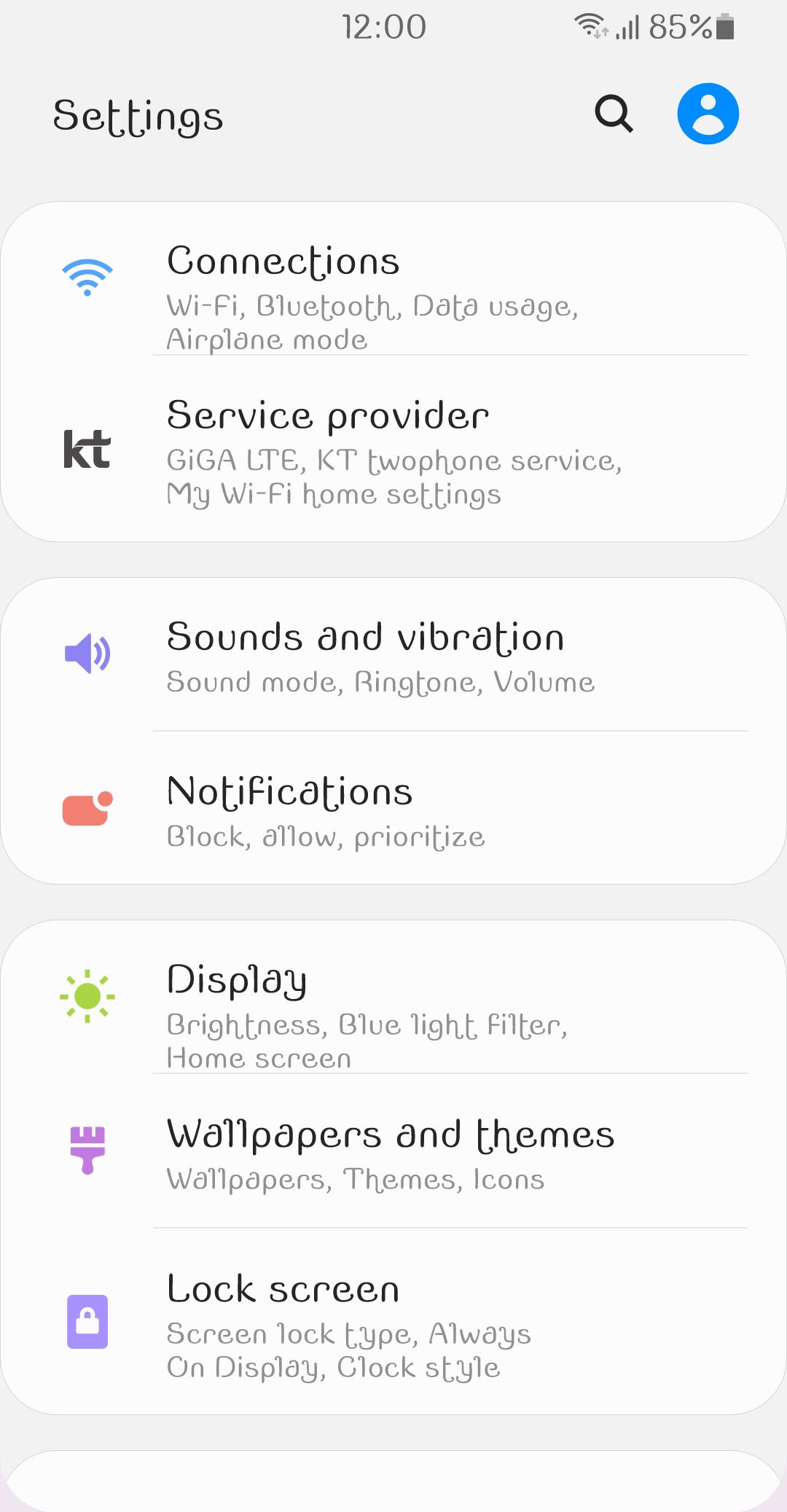An image displaying a smartphone settings screen with a light gray background is depicted. At the top, the status bar shows the time as "12", full Wi-Fi signal strength, and an 85% battery level. On the left, the word "Settings" is displayed, while a magnifying glass icon appears on the right. Below the status bar, the screen is divided into various sections:

1. A blue circle with a white dotted head and shoulders icon symbolizing a user account or profile.
2. A white rounded box titled "Connections" with subsections: Wi-Fi, Bluetooth, data usage, and airplane mode. Below this is a gray line followed by "Service Provider" details indicating the provider as KT, along with "Giga LTE KT" for service specifics.
3. "My Wi-Fi home settings" is listed next.

Further down, another white box features a purple sound icon. The section is labeled "Sounds and Vibrations" containing options like sound mode, ringtone, and volume.

Next, an orange partial square with an orange dot beside text reading "Notifications" categorized into block, allow, and prioritize appears. Following this, there is a green spacer and more gray spacing.

A white rounded square with a green sun icon denotes the "Display" settings, which include brightness, blue light filter, and home screen options.

Lastly, a purple paintbrush icon leads to "Wallpapers and Themes", where one can adjust wallpapers, themes, and icons. Below that, a purple box with a white padlock icon indicates "Lock Screen" settings covering screen lock type, always-on display, and clock style. Gray spacing follows, ending with another white circle.